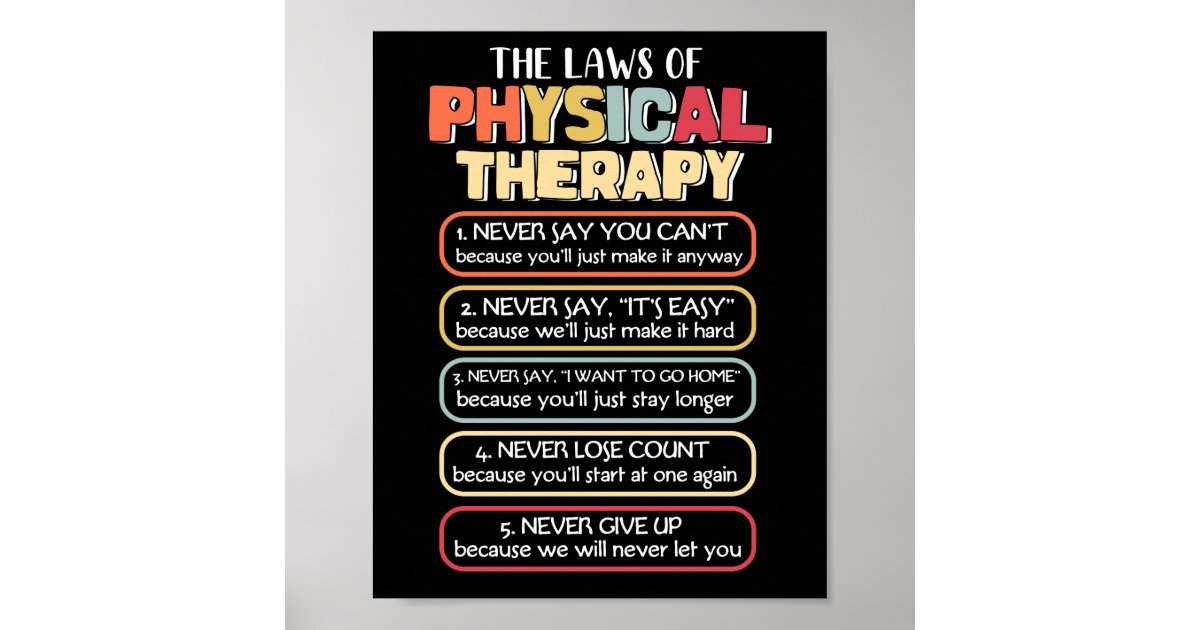This image portrays a detailed poster with a solid medium gray background that gradually transitions from darker on the right to lighter on the left. In the center of this backdrop sits a black vertical rectangle, resembling a poster. At the top of the poster, the title "THE LAWS OF PHYSICAL THERAPY" is prominently displayed in all caps white text. 

The word "PHYSICAL" is colorfully written in block style, all-caps letters: "PH" in orange, "YS" in tan, "IC" in blue, and "AL" in red. Below that, "THERAPY" appears in light tan, block letters. 

Under the title, there are five distinct sections, each bordered by a different color and containing white text. The first section is framed in orange and reads:
1. NEVER SAY YOU CAN’T
   because you’ll just make it anyway. 

The second section, bordered in yellow, states:
2. NEVER SAY IT’S EASY
   because we’ll just make it hard.

The third section, highlighted with a blue border, advises:
3. NEVER SAY I WANT TO GO HOME
   because you’ll just stay longer.

The fourth section, enclosed in beige, warns:
4. NEVER LOSE COUNT
   because you’ll start at one again.

The fifth and final section, with a red border, declares:
5. NEVER GIVE UP
   because we’ll never let you.